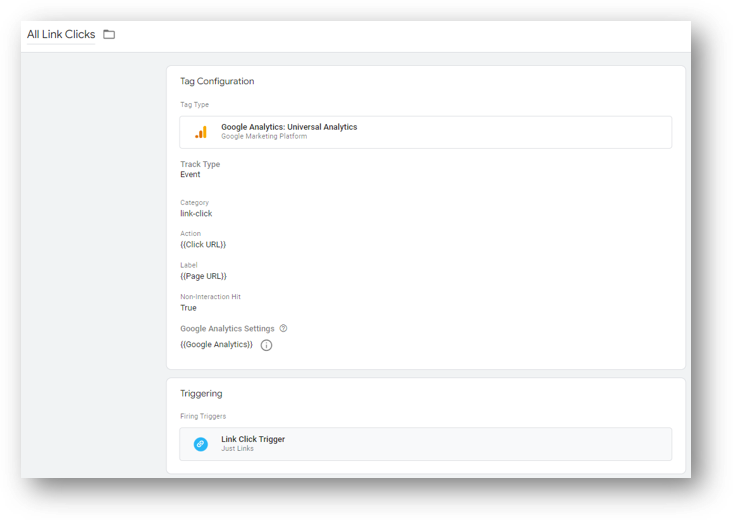The image displays a screenshot of a computer screen showcasing various sections related to link clicks configuration. At the top, the screen features a heading labeled "All Link Clicks" within a white area that includes an icon resembling a file folder. Below this, there is a section titled "Tag Configuration," followed by another labeled "Tag Type."

Dominating the center of the image is a long, slim white rectangle bordered in gray. Inside this rectangle, three orange and red bars—resembling a bar graph—are situated. Alongside these bars, bold text reads "Google Analytics: Universal Analytics," and beneath that, in gray print, it says "Google Marketing Platform."

Further down the screenshot, the section labeled "Track Type" is visible, with "Event" listed directly underneath it. Subsequent fields include "Category," which shows "Link - Click," followed by "Action," noted as "Click URL" in parentheses. Then comes "Label," enclosed in double parentheses as "(Page URL)."

At the bottom of the image, there is a final section that mentions "Link Click Trigger." This is accompanied by the description "Just Links" and features a blue circle icon.